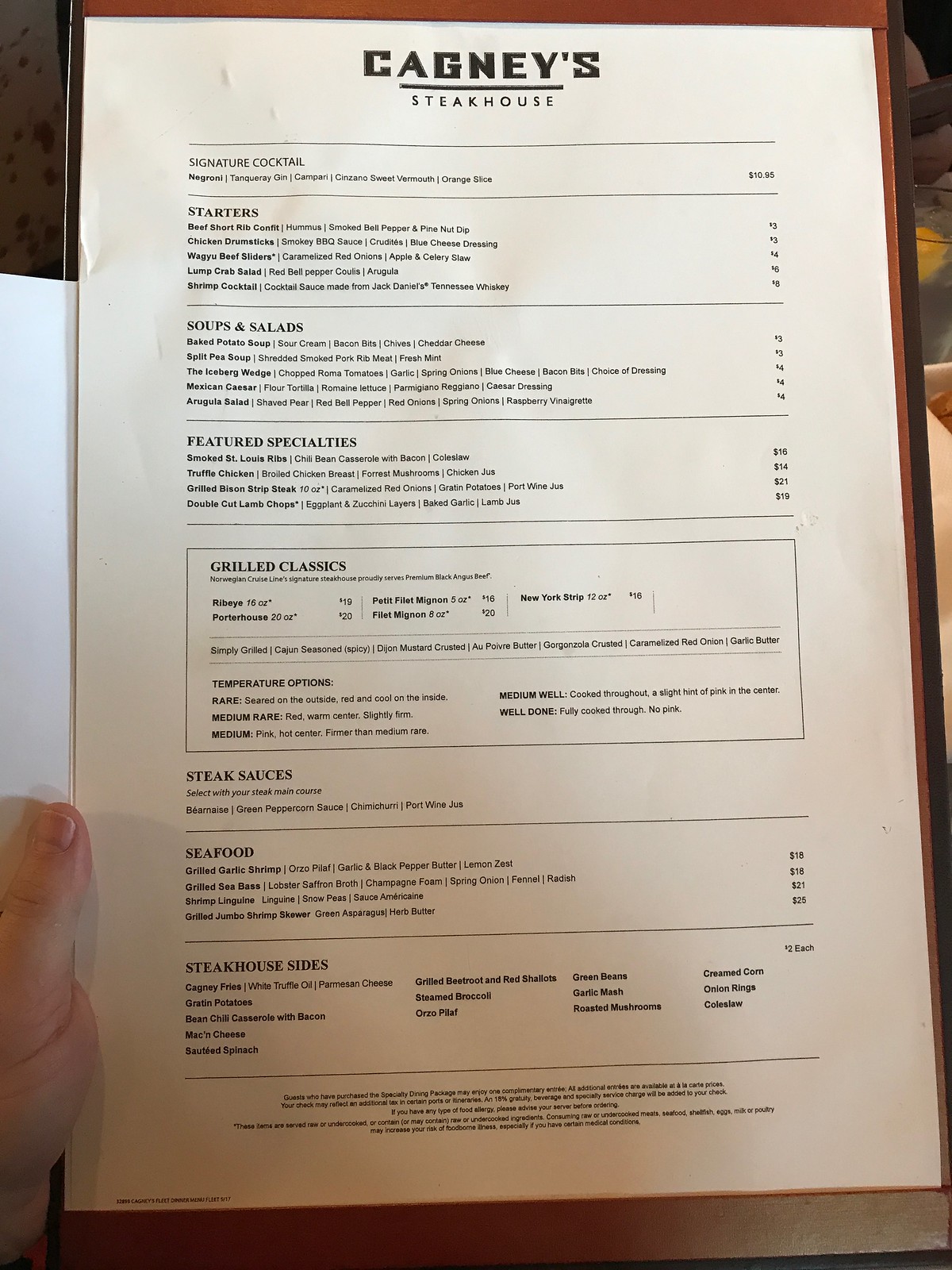The image features an A4-sized menu for Cagney Steakhouse, printed on an off-white sheet of paper. The menu layout is well-organized, with clear and legible text. At the top, "Cagney Steakhouse" is prominently displayed in large letters, catching the viewer's attention immediately. 

The sections of the menu include "Signature Cocktails," "Starters," "Soups and Salads," "Featured Specialties," and boxed in the center are "Grilled Classics." Following these, the menu lists "Steak Sauces," "Seafood," and "Steakhouse Sides." Each menu item comes with a detailed description and prices listed in dollars. 

Despite some small print at the bottom being hard to discern, the overall presentation is neat and appealing. The image itself shows a person holding the menu with their left hand, with their thumb visible on the left edge of the menu. The background behind the menu adds to the aesthetic, creating a sense of context and atmosphere.